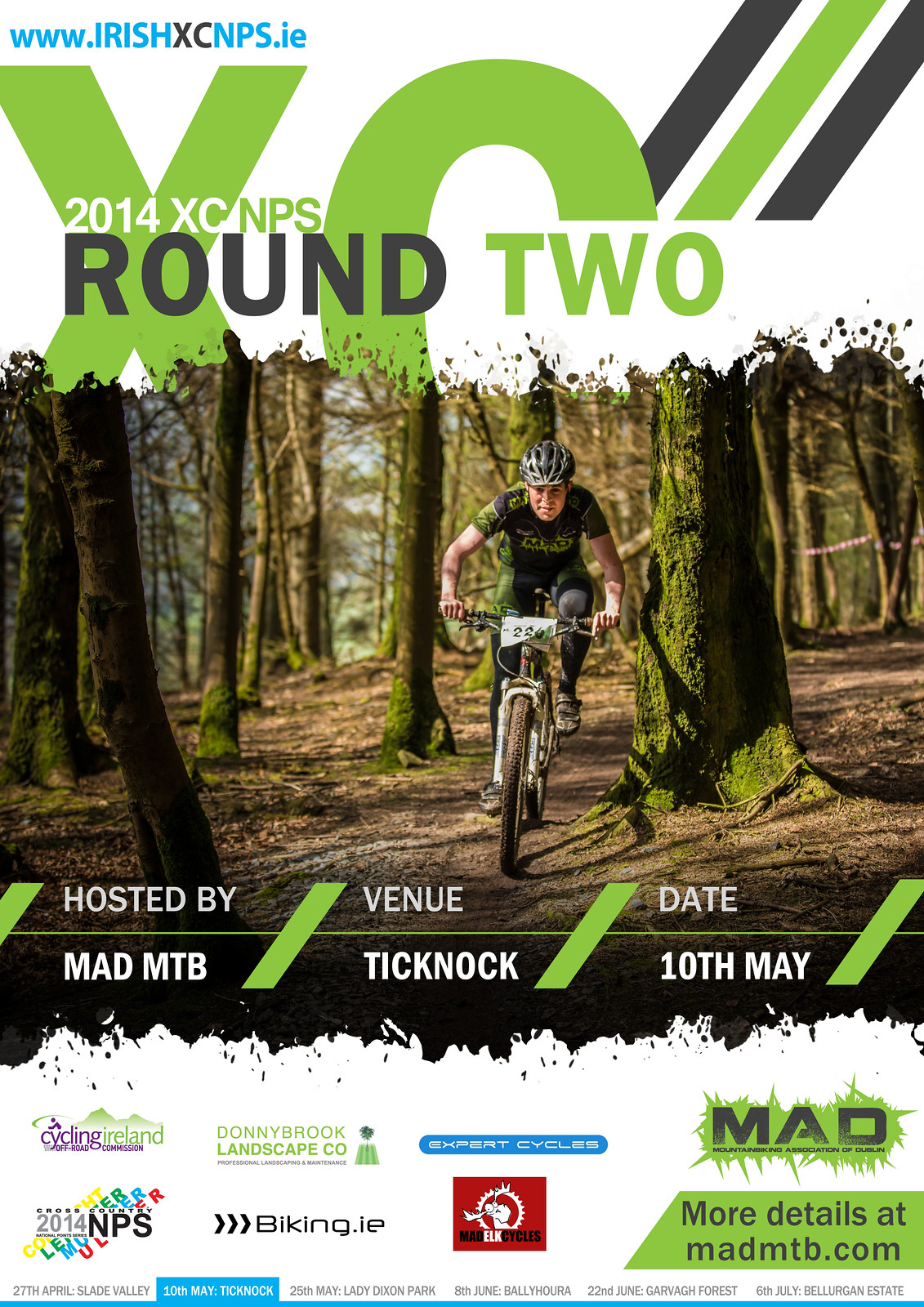The rectangular image appears to be a detailed advertisement for a mountain biking event. At the center, it features a dynamic photo of a mountain biker racing through a wooded trail on a dirt and rocky surface, suggesting he is participating in a competitive race. The biker is dressed in a black and green cycling shirt and pants, complete with a helmet, and his bike has a black and white race number on the handlebars. In the background, trees and a bit of sky are visible, reinforcing the outdoor setting, which appears to be during the daytime.

Across the top of the image, the text "2014 XC NPS Round 2" is prominently displayed, with a website address, www.irishxcnps.ie, written in blue above it. Information further indicates that the event is hosted by MAD-MTB at the venue Ticknock on the 10th of May. 

Toward the bottom of the image, on a white background, there are logos and names of various sponsors such as biking.ie, Donnybrook Landscaping Company, and others, indicating their support for the event. Additionally, it directs viewers to madmtb.com for more details. The overall design combines multiple colors, including white, green, black, light blue, brown, light green, purple, and red, making it visually engaging and informative.